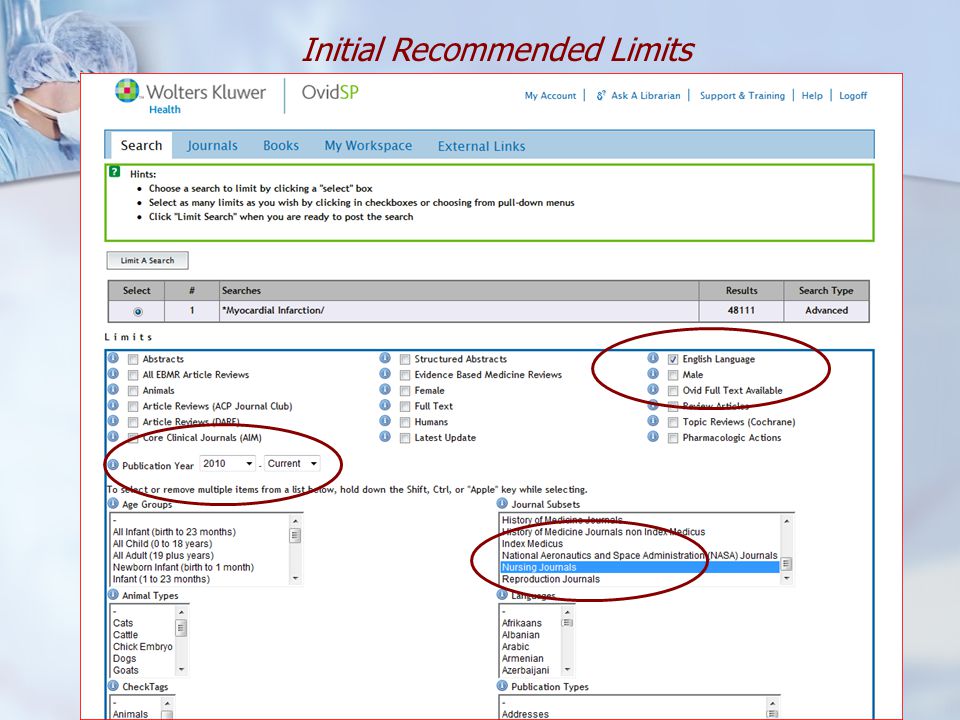This image features a soft, light blue background with a partial profile view of a healthcare professional, identifiable either as a nurse or a doctor. The individual is equipped with a hairnet, surgical mask, and surgical gown, embodying a sterile and professional environment. Superimposed over this backdrop is text from a digital interface that reads, "Initial recommended limits Wolters Kluwer Health." Below this, there are instructions stating: "Choose a search to limit by clicking a select box. Select as many limits as you wish by clicking in checkboxes or choosing from pull-down menus. Click 'Limit Search' when you're ready to process the search."

Highlighted prominently are three distinct red circles, each encompassing different sections of the text interface. The first circle emphasizes "care clinical journals AIM publication year 2010 current." The second circle draws attention to "Index Medicus, National Aeronautics and Space Administration, nursing journals, and reproduction journals." Finally, the third circle encircles "English languages, male, over, full text available." These markings seem to indicate specific selections or settings within a medical or research database interface.